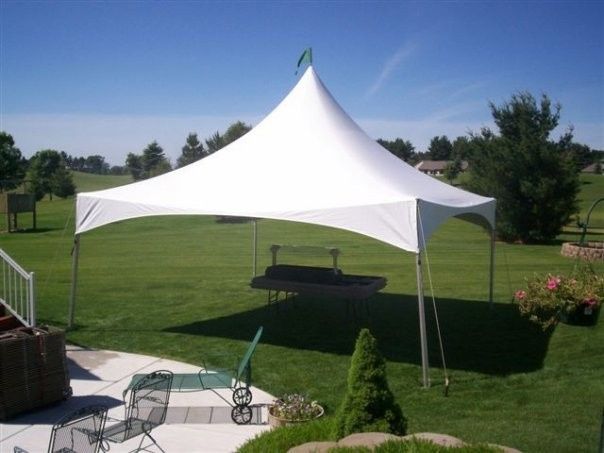The photograph showcases a serene backyard setting bathed in daylight under a clear blue sky. At the center of this verdant scene is a large canopy with a white tarp, supported by gray poles and secured with stakes and ropes, providing shade for a small table beneath it. The surrounding environment features well-manicured green grass and various pieces of outdoor furniture, including two simple black lawn chairs and a green metal lounging chair, which rest on a gray concrete patio to the left of the canopy. 

To the bottom center is a meticulously trimmed small green tree, while directly to the right of the canopy hangs a pot of blooming flowers, introducing bursts of pink against the greenery. Nearby, a circular arrangement of red bricks likely indicates the presence of a well or decorative stone feature. The leftmost side of the image reveals a portion of a white-railed staircase leading to the patio. 

In the far background, an expansive field dotted with trees stretches out, and a glimpse of a small distant house with a gray roof can be seen just above and to the right of the canopy. The overall ambiance suggests a peaceful outdoor space, possibly prepared for a relaxed gathering or afternoon barbecue.